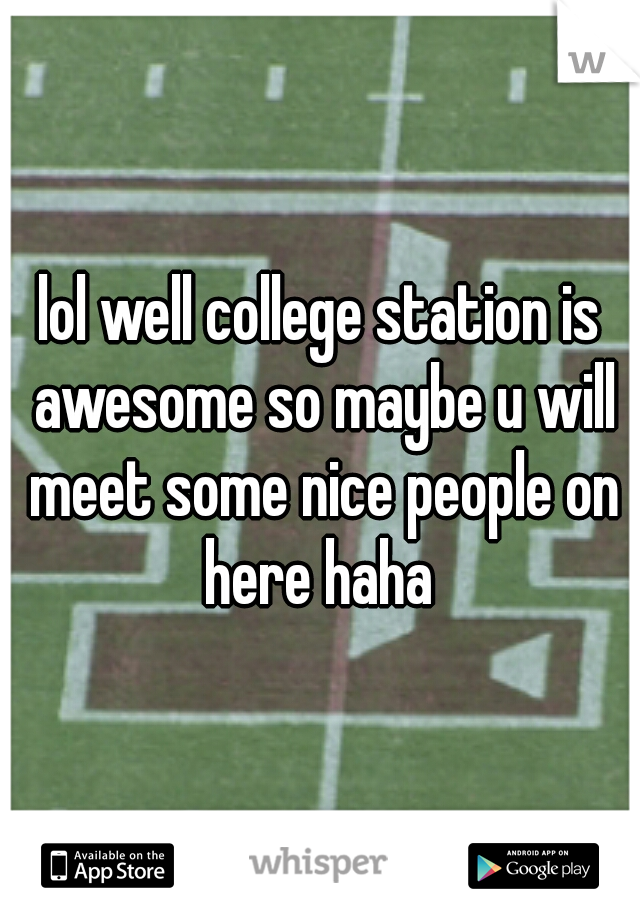The image showcases a segment of a football field dominated by a large Texas A&M "T" logo. The "T", noticeably clear yet flanked by hints of the adjacent letters 'A' and 'M', is large, red, and outlined in white, partially visible with the 'A' on the left and the start of the 'M' on the right. In the background, the green football field is detailed with white dashes and other field markings, possibly the 50-yard line which is indicated by a vertical white line running down the center. Overlaying the logo, there's white text in four lines that reads, "LOL, well, College Station is awesome, so maybe you will meet some nice people on here, haha." The text is prominently centered over the "T". At the top right corner is a capital "W" representing Whisper. Towards the bottom, there is light gray text that reads "Whisper". Below the image, there are store icons; on the left side, a little rectangular icon says "Available on the App Store" with the Apple logo, while on the right, another icon says "Google Play" with a triangle play sign and "Android app on Google Play".